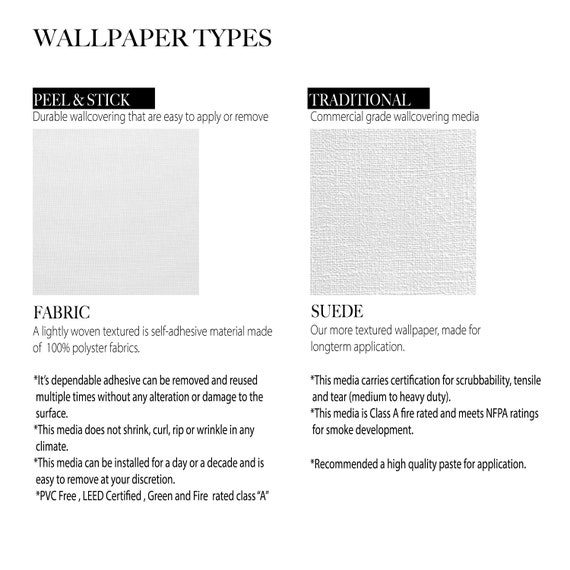The image displays a detailed comparison of two different types of wallpaper, presented in black and white. On the left, under the heading "Peel and Stick," there is a sample of fabric wallpaper described as a lightly woven, self-adhesive material made of 100% polyester. This fabric wallpaper is praised for its dependable adhesive, removable and reusable multiple times without causing any damage to the surface. It does not shrink, curl, rip, or wrinkle in any climate, and can be installed for as short as a day or as long as a decade with easy removal at any time. It is PVC-free, lead-free, environmentally friendly, and fire-rated as Class A. On the right, under the heading "Traditional," there is a sample of suede wallpaper, described as a more textured, commercial-grade wall covering medium made for long-term application. This wallpaper is certified for scrubability, tensile strength, and tear resistance, making it suitable for medium to heavy-duty use. It also meets Class A fire rating and NFPA ratings for smoke development, with a recommendation for the use of high-quality paste during application. Both wallpaper samples are displayed in light gray squares, with the suede sample appearing slightly more textured than the fabric. Below each sample, user reviews highlight the reliability and durability of these wallpapers, reinforcing their high quality and performance standards.